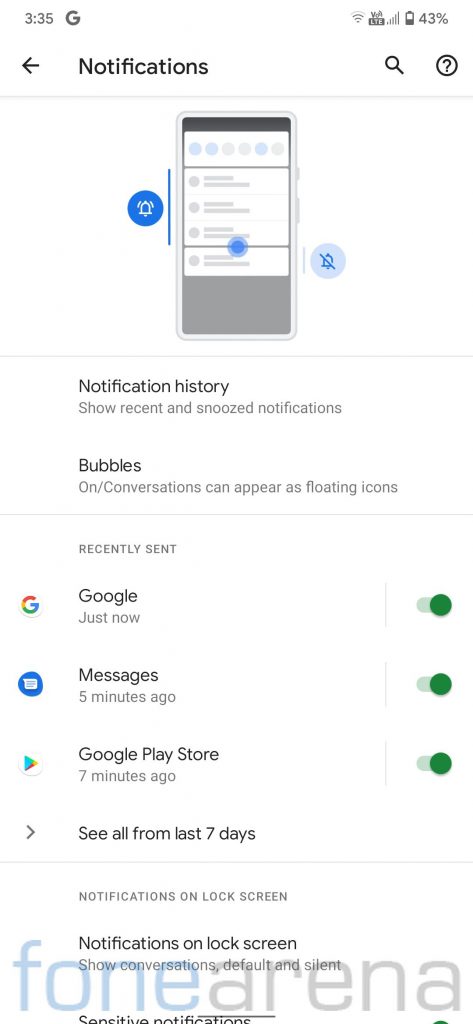The image features a smartphone interface displayed against a white background. At the top of the screen, the time shows 3:25 PM, with a notification icon in the "G" symbol for Google at 43% battery. The navigation bar includes an arrow pointing left, a search magnifying glass icon, and a circle with a question mark.

The phone's display provides a detailed view of notification settings. On the upper left, there's a blue circle with a white notification bell, signifying active notifications. Adjacent to it, a gray circle with a bell and a slash indicates muted notifications. An option highlighted in blue shows "Notification History," offering the ability to "Show recent and snoozed notifications." Below this, a toggle for "Bubbles," which enables conversations to appear as floating icons, is activated.

Recently sent notifications are listed below:
- "Google" with a green circle, received just now, toggle bar set to "on."
- "Messages" received five minutes ago, toggle bar set to "on."
- "Google Play Store" received seven minutes ago, toggle bar set to "on."

A link saying "See all from last seven days" is also present. At the bottom, there is a mention of "Phone Arena," with "Phone" in blue text and "Arena" in gray, suggesting a source or category.

The settings section further includes options for "Notifications on lock screen," which can show conversations either defaulting or in silence.